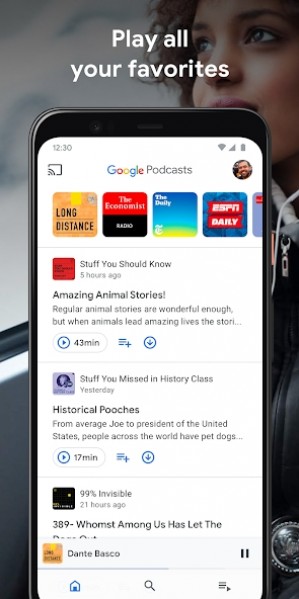A vibrant image portrays a scene from Texas with various favorite shows playing in the background. In the foreground, a person with curly hair is slightly out of focus, adding a dynamic depth to the picture. The person's smartphone screen is clearly visible, displaying the time as 12:30 PM with full Wi-Fi signal, and battery. They are using Google Broadcast, and their profile picture is prominently shown. The screen indicates a long-distance call with an exponential symbol. The phone interface features a mix of blue and yellow colors. Among the displayed items are icons and headers such as "Stuff You Should Know," "The Amazing," and "Stuff You've Missed in History Class." These highlight a variety of intriguing shows and podcasts that tackle everything from amazing animal stories to historical events. One of the shows has a duration of 43 minutes, and topics range from pet dogs of the U.S. Presidents to subtle design elements, indicated by the "99% Invisible" icon. Dante Basco's name appears alongside an orange square symbol. A blue house icon is placed on the left of the screen, contributing to the colorful and information-rich nature of the scene.